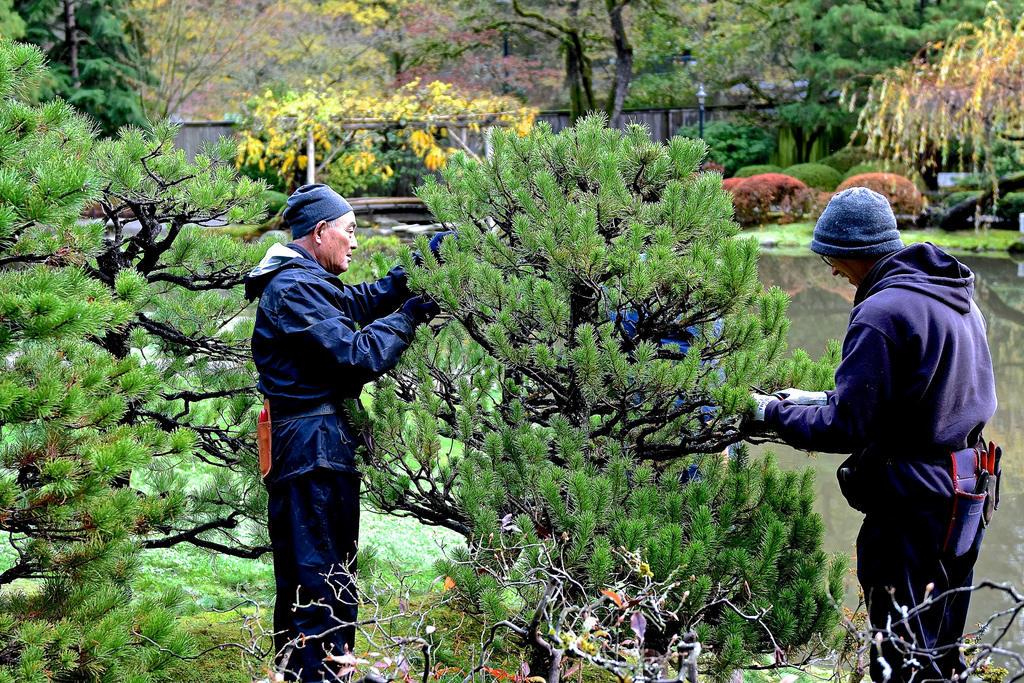In this beautifully sharp and detailed photograph, two men are captured meticulously working in a well-kept garden, giving a strong impression of a serene Oriental setting. Both men are dressed in dark blue work attire, including hoodies and caps. The man on the left, wearing a stretch cap and a blue jacket with a hood, is seen reaching into a large evergreen bush with two gloved hands, his waist adorned with a leather holster holding pruning tools. The man on the right, who sports a knit winter cap, glasses, and lighter gloves, appears to be wielding a pair of clippers while his belt holds additional holsters. They both are standing on either side of a sizeable pine tree, about six or seven feet tall, which they are carefully pruning. The garden around them is lush with various greenery, including another similar-sized pine tree, weeping willows, and a variety of bushes and evergreen plants. In the mid-ground, there's a small pond bordered by more bushes and willows, and further back, a wooden bridge crosses a waterway, enhancing the tranquil, manicured landscape. The entire scene conveys a feeling of precision and peace, reminiscent of traditional Japanese gardens.